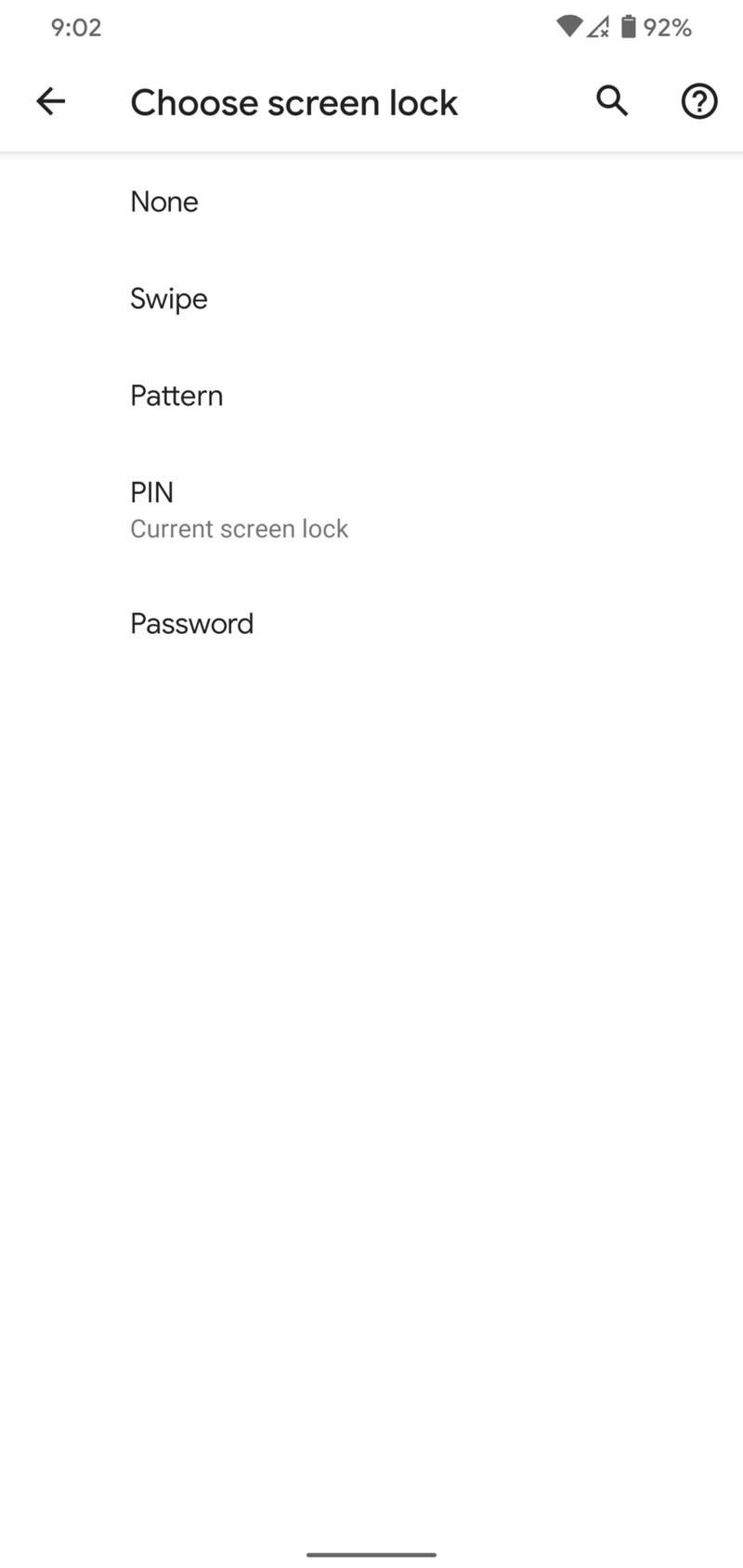The image displays a printout of a digital device screen related to a password entry interface. At the top left, there is a timestamp reading "9:02" with a downward-pointing arrow directly below it. To the right of the timestamp, several icons are visible, along with a battery indicator showing a 92% charge.

In the center of the screen, the words "Choose Screen Lock" are prominently displayed in dark gray font on a white background. These words are accompanied by an hourglass icon and a question mark enclosed in a circle. This section is the focal point of the image due to the larger font size.

Beneath this heading, the printout lists different screen lock options from left to right: "None," "Swipe," "Pattern," "Pen," and "Current Screen Lock." The last option listed is "Password," indicating the current screen lock method. There is a prompt suggesting that information can be entered, although no data has been inputted yet.

Additionally, there is a faint, barely-visible line at the bottom of the image, suggesting it may be a copy of a copy. The overall layout is clean, and the text clarity indicates the primary focus is on selecting and managing screen lock options.